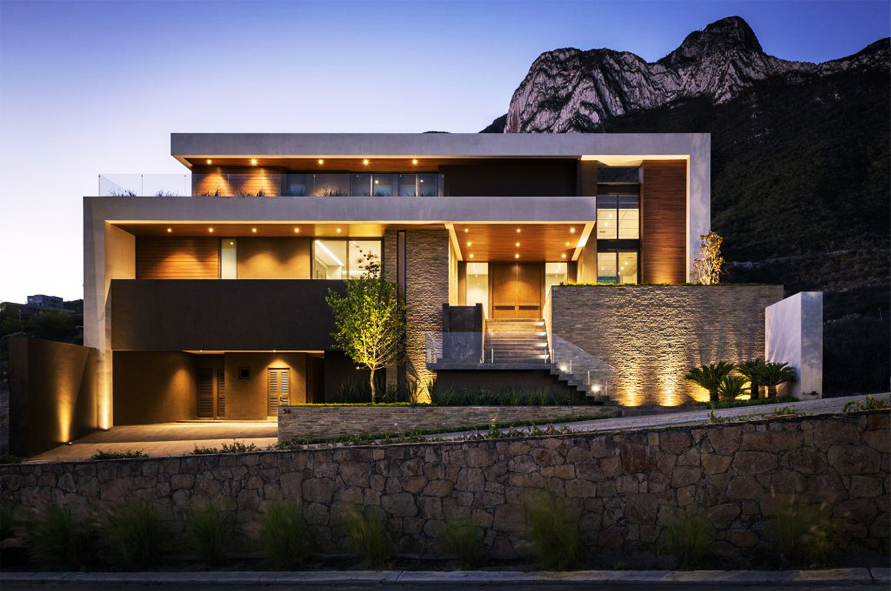This color photograph captures the exterior of a striking, modern-style, three-level home at dusk. The house, positioned at the base of a large, rocky mountain with snow-capped peaks in the background on the right, features a boxy architectural design with a predominantly wooden exterior. A stone wall serves as the driveway's base in the foreground, supporting the driveway above it. 

The ground level boasts an entry door to the left and is adorned with warm wooden textures. A large wooden balcony spans across the second level, accessible via an elegant staircase with a glass divider. The double brown wooden front doors, located on the second level, are highlighted by recessed lighting above. Adjacent to these doors is a striking large stone wall flanked by a white marble wall accent, surrounded by baby palm trees accentuated with up lighting.

The third level, slightly set back from the roofline, includes another glass balcony. Prominent floor-to-ceiling windows extend across both the second and third levels on the right side, offering glimpses inside the illuminated interior. The surrounding landscape is tastefully lit with track lighting, and the front yard is adorned with a small tree and various shrubs. The dark blue sky hints at the setting sun, completing this picturesque scene of contemporary elegance.